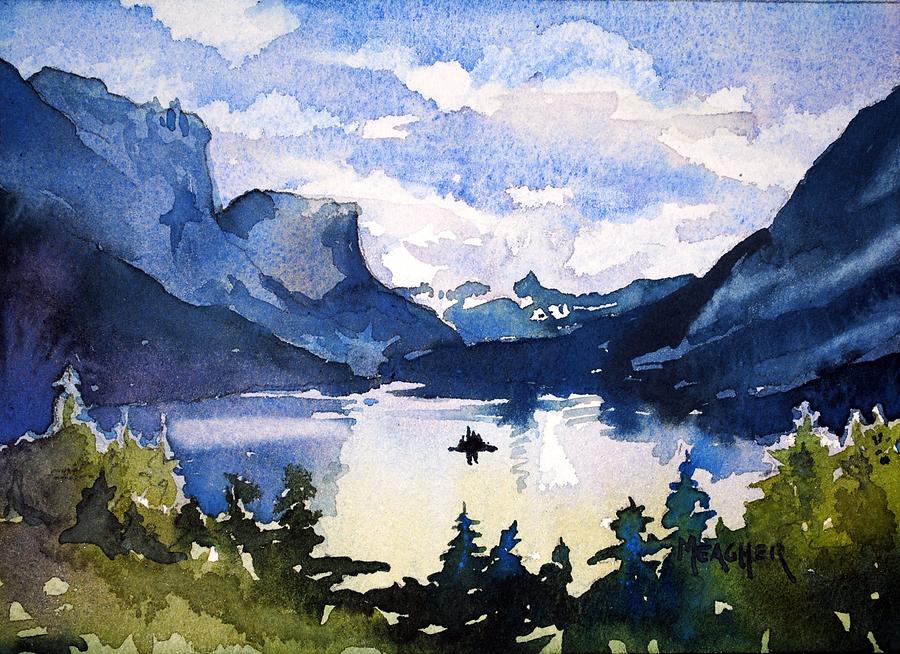This painting, an impressionistic watercolor by an artist named Meagher, beautifully depicts a serene lakeside scene. The center of the composition features a tranquil lake bordered by blue hills and mountains, with a fluffy blue and white sky overhead. The lake itself showcases a blend of colors, with areas of yellow, white, and shades of blue, suggesting the mingling of reflections and water. In the middle of the lake resides a black object that could be interpreted as either a boat with figures or a small tree-covered island. The foreground is adorned with green pine trees, varying in hues of light green, dark green, and blue, rendered in an impressionistic style, focusing on outlines and colors rather than intricate details. The overall effect is one of soft, dreamlike beauty, characteristic of watercolor’s fluidity. The artist’s signature, "Meagher," is prominently placed on the bottom right corner of the painting.